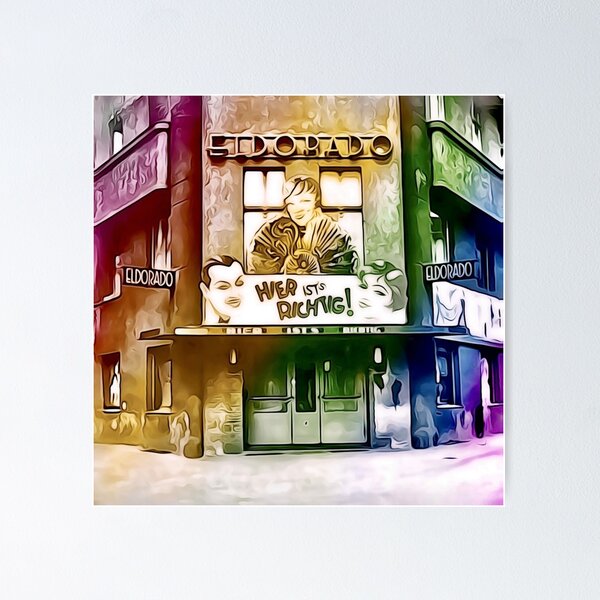This image is a watercolor-style, possibly computer-generated depiction of a corner storefront, reminiscent of an entertainment venue such as a nightclub, movie theater, or cocktail bar. The building features a faded rainbow gradient, blending hues from pink through purple. Mounted on a light-colored wall, the façade displays a vintage, 1920s-1930s flapper-style aesthetic. At the top, the marquee prominently reads "El Dorado" in an old-style movie-theater-type font. Below this central sign, there's an image of a woman holding a fan, evocatively styled from the early 20th century. Flanking either side of the entrance are slanted walls with black signs, each reiterating the “El Dorado” name. Just below these signs, the doorway itself is centrally located. Below the central image of the woman, on the left, is a man with slicked-back hair and a thin mustache, and on the right is a woman with styled hair from the same era, adding to the vintage vibe. Additionally, a marquee in German with the text "Hier ist Richtig!" sits near the entrance, underscoring the thematic blend of old-world charm and modern artistic representation.